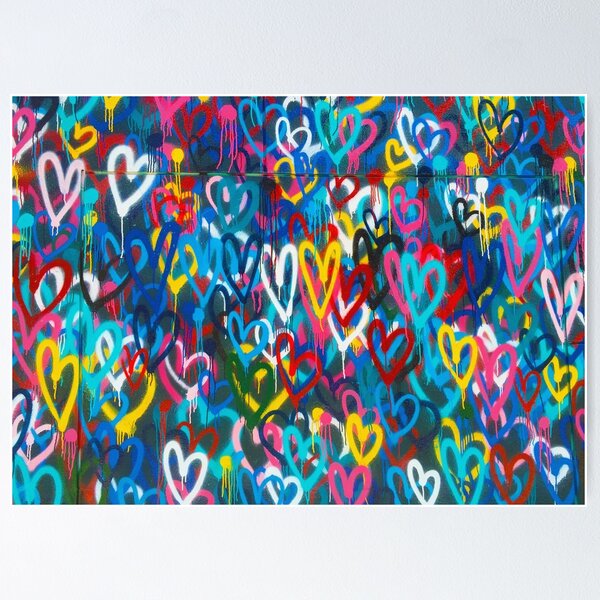This vibrant, modern piece of art, reminiscent of graffiti, is a rectangular painting framed in a narrow silver border. The artwork is entirely filled with hand-drawn hearts, overlapping and clustered together, creating a dense tapestry of color and form. The hearts range in hues from neon yellow, blue, and pink, to darker tones of green and blue, with occasional white and red hearts standing out against a barely visible dark green background. The paint from the hearts, some solid, some merely outlined, slightly drips, adding to the graffiti effect. The hearts—varying slightly in shape but similar in size—cover the entire canvas in a lively, chaotic yet visually striking manner, where every corner pulsates with the energy of its bright, dripping colors.